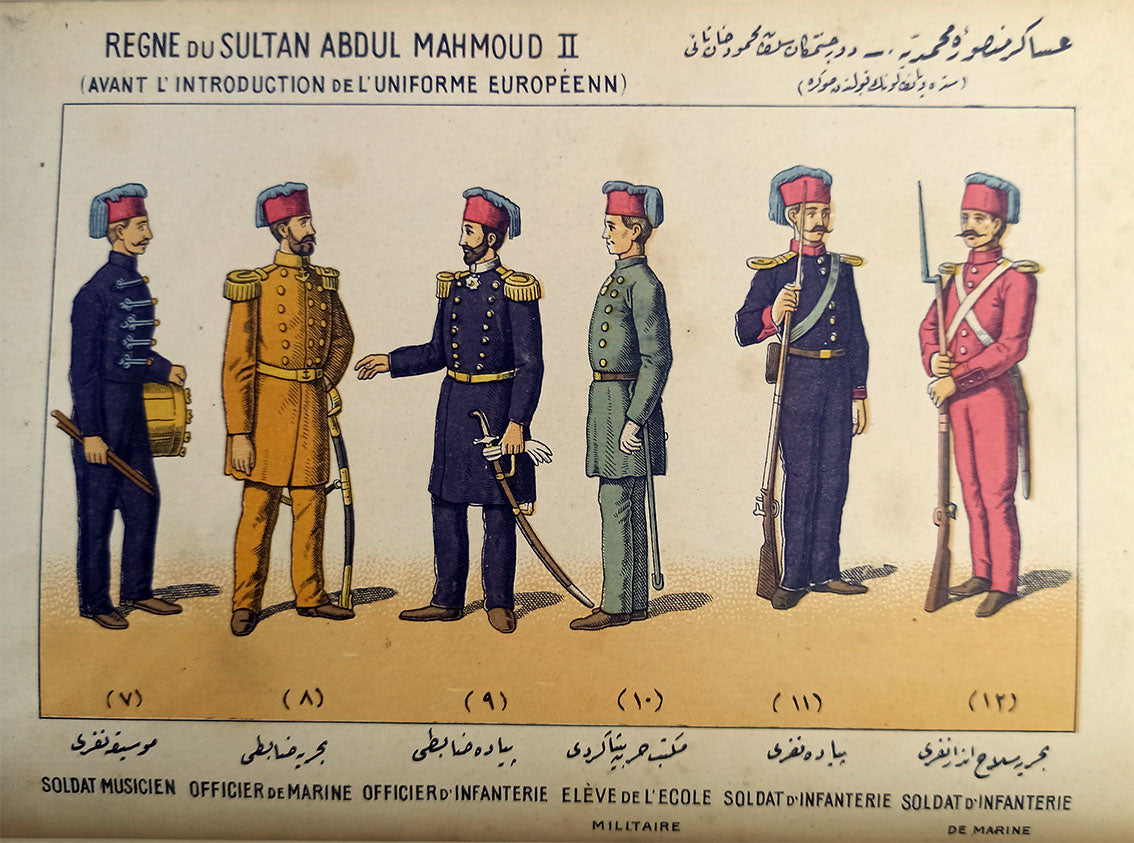The image shows a colorful illustration set against an ivory background, enclosed by a black rectangular outline. At the center, there are six men standing in a row, each in different colored uniforms, including blue, gold, green, pink, and orange. These men appear to be soldiers, wearing coordinated hats that are red with blue tops. Their uniforms are ornate with gold shoulder pads, brass buttons, and gold sashes around their waists. Alongside their uniforms, some soldiers are holding rifles or swords, while one on the far left has a drum and drumstick. The top of the illustration features text in a different language, indicating "Regni du Sultan Abdul Mahmoud II" and "Rejner Do Sultan Abdul Mahmud Do Avant L Introduction D D L Uniform European," with additional names written at the bottom identifying each figure as various types of military personnel, such as "Soldat Musician," "Officer D Marine," "Officer D Infantry," "Leve D Likol," and "Soldat D Infantry." The scene is clearly lit and vibrant, capturing a detailed and lively depiction of historical soldiers.